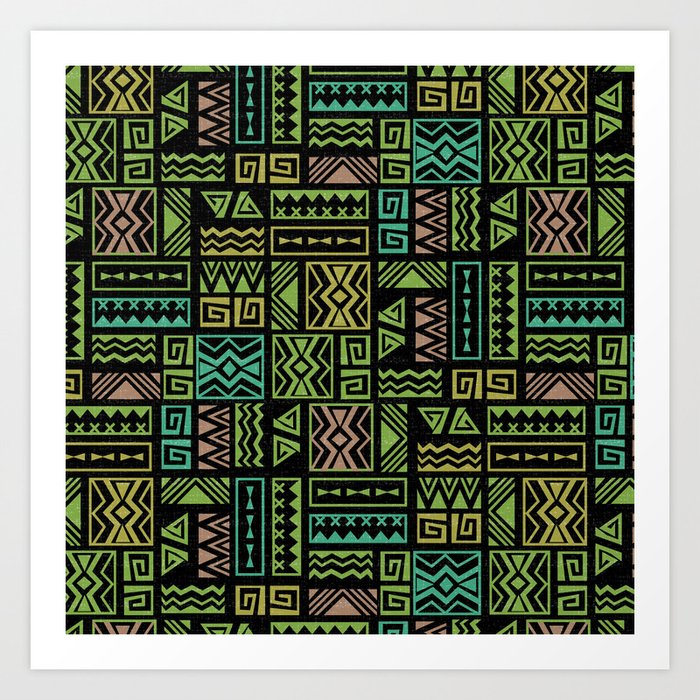The image is a square piece of art framed by a light gray outer border and a white mat. The artwork itself features a black background with an array of colorful shapes, including triangles, spirals, zigzags, and bowtie-like designs, which evoke an African tribal aesthetic. These shapes are predominantly green, red, blue, pink, and yellow, and are arranged in a grid-like pattern with variously sized and shaped squares and rectangles. The vibrant geometric patterns are separated by black lines, providing a striking contrast against the dark backdrop.